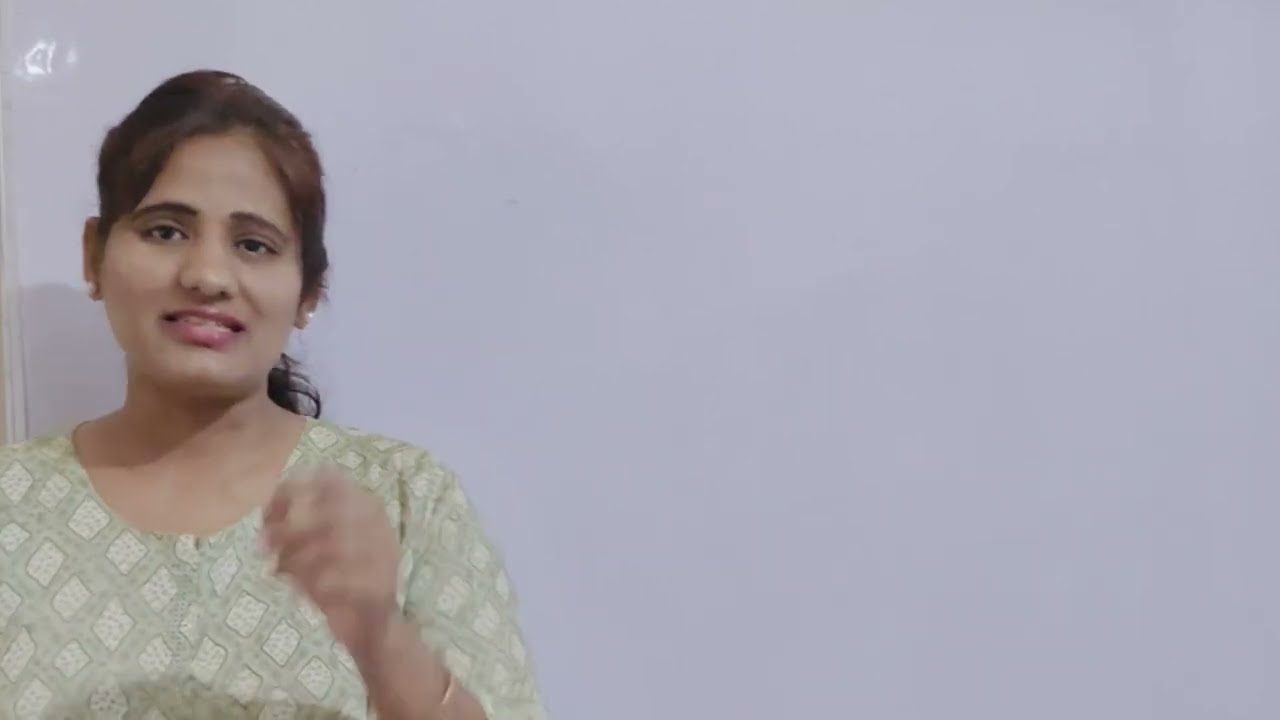The image features a woman with distinctive Indian features positioned towards the far left side of the frame, set against a light gray to bluish background with ample empty space to the right. Above her head, there's a white spot that appears to be a reflection of light, along with a logo resembling a house in the upper left corner, hinting that this could be a screenshot from a video, podcast, or social media profile picture. She has olive complexion, dark brown eyes, and dark eyebrows, and her dark hair is pulled back in a ponytail. She is smiling directly at the camera, wearing red lipstick and pearl earrings. Her attire includes a green top with white diamond shapes adorned with green specks. On her left wrist, she sports a bracelet, and her left hand, slightly blurry as if in motion, is raised with fingers loosely closed.